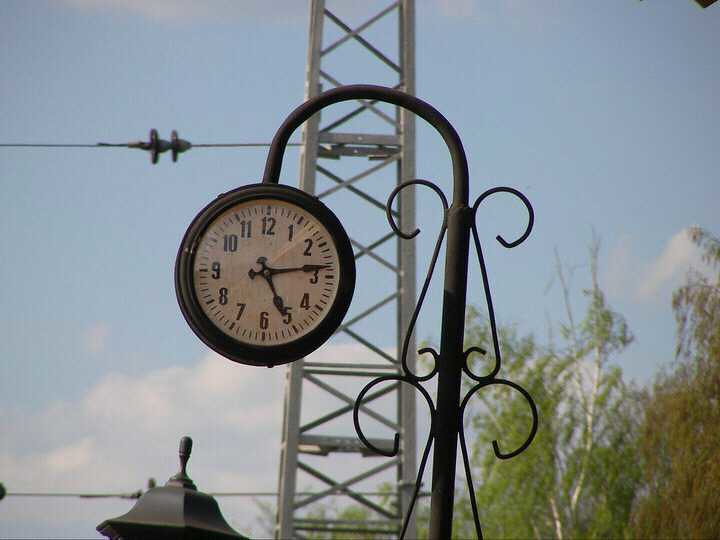This photograph captures an ornate outdoor clock hanging from a gracefully designed wrought iron pole that resembles an inverted U. The pole features intricate curlicue embellishments, adding to its decorative elegance. The round clock, bordered in black, presents a white-and-gray face with standard black numerals and hands. The time displayed is approximately 5:14. The image quality is pixelated, but the details are discernible. Behind the clock, a large metal structure with two horizontal wires stretching out from it is visible. To the left at the bottom of the photograph, the top of a bronze-colored cupola is apparent. Further in the background, the tops of leafy trees can be seen against a backdrop of a clear blue sky dotted with a few fluffy white clouds.